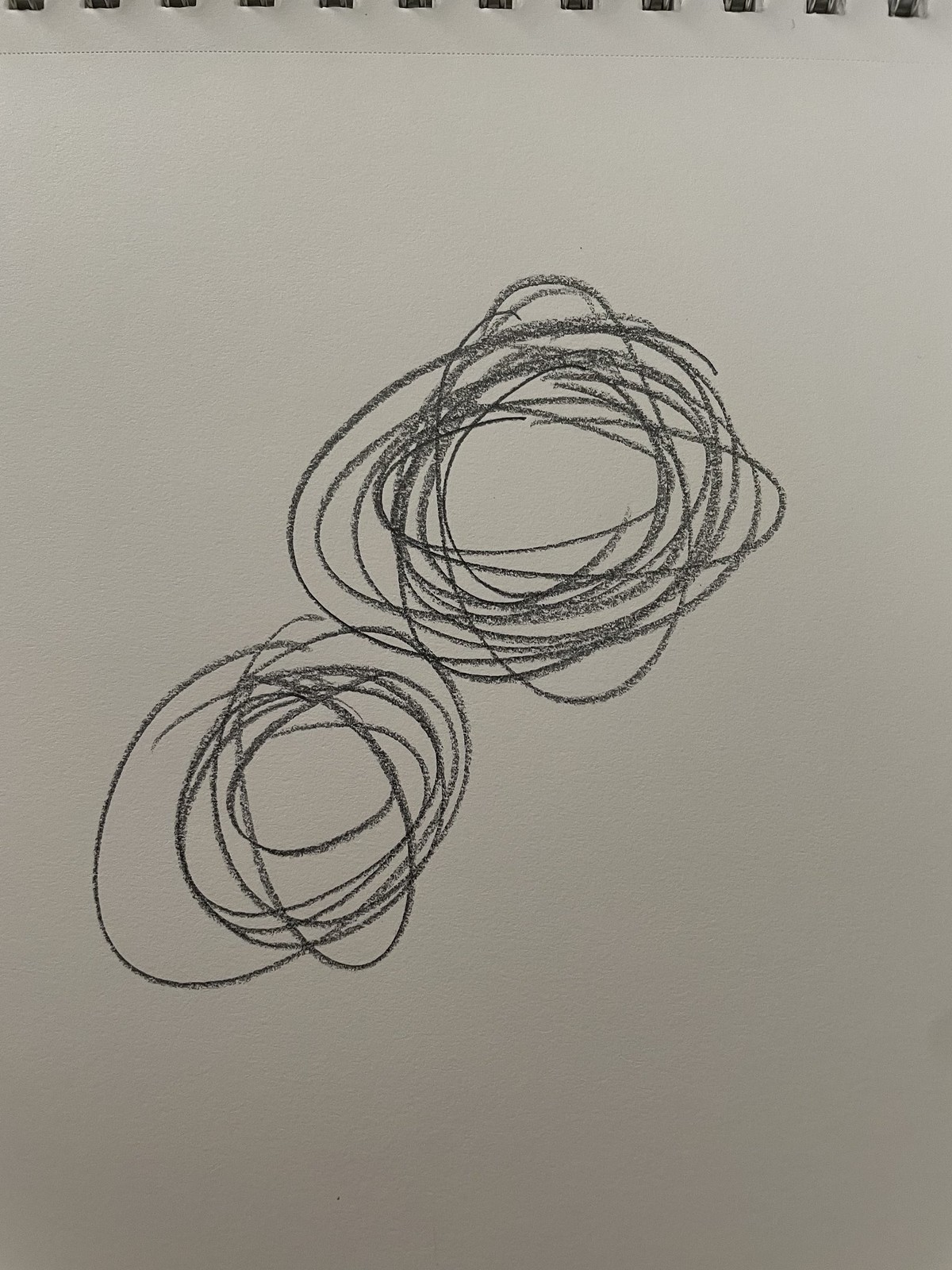The image depicts a piece of high-quality, thick white paper from an art binder. The top edge of the paper showcases a perforated line, facilitating easy removal from the binder. This binder is held together by twelve visible metal rings. Dominating about one-third of the page are two scribbles, likely drawn with crayon given their waxy finish. These scribbles consist of elongated oval shapes layered on top of each other in various directions, creating intricate, solar system-like patterns. The first and larger scribble occupies an upper central position, while the second, smaller scribble sits below and slightly to the left of the first, positioned in a south-west direction.